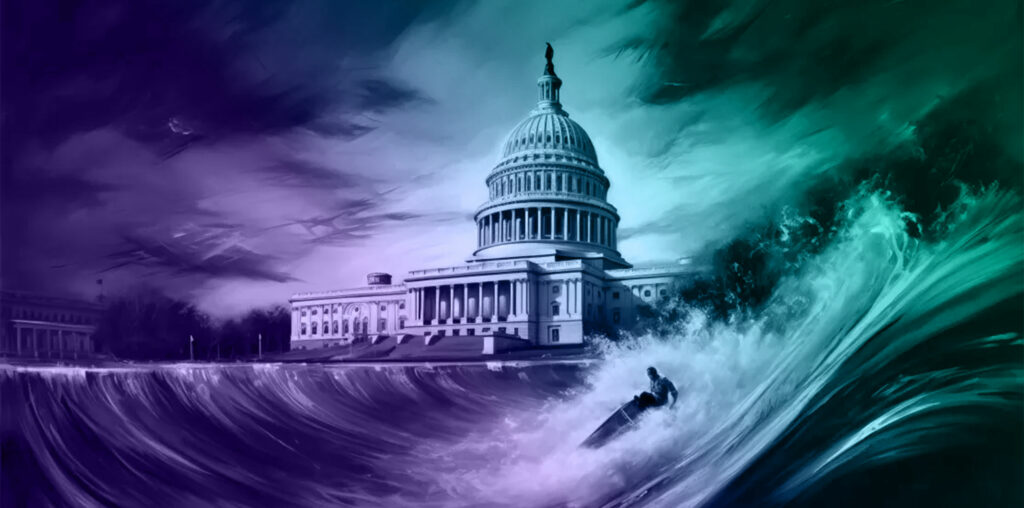This is a rectangular digital art piece featuring the US Capitol building in the background, centered on the image. The left portion of the image is primarily in shades of purple that become darker as they reach the edge, while the right side transitions to a darker green and blue palette. Above the Capitol, the sky appears stormy with black, purple, and green highlights. In the sea, to the right of the Capitol, there is a large, wild wave with crashing whitecaps. A single person is seen riding this tumultuous wave on a surfboard, adding a dynamic and surreal element to the scene. Despite the digital creation, the artwork has a hand-drawn quality, enhancing its unique and dramatic appearance.